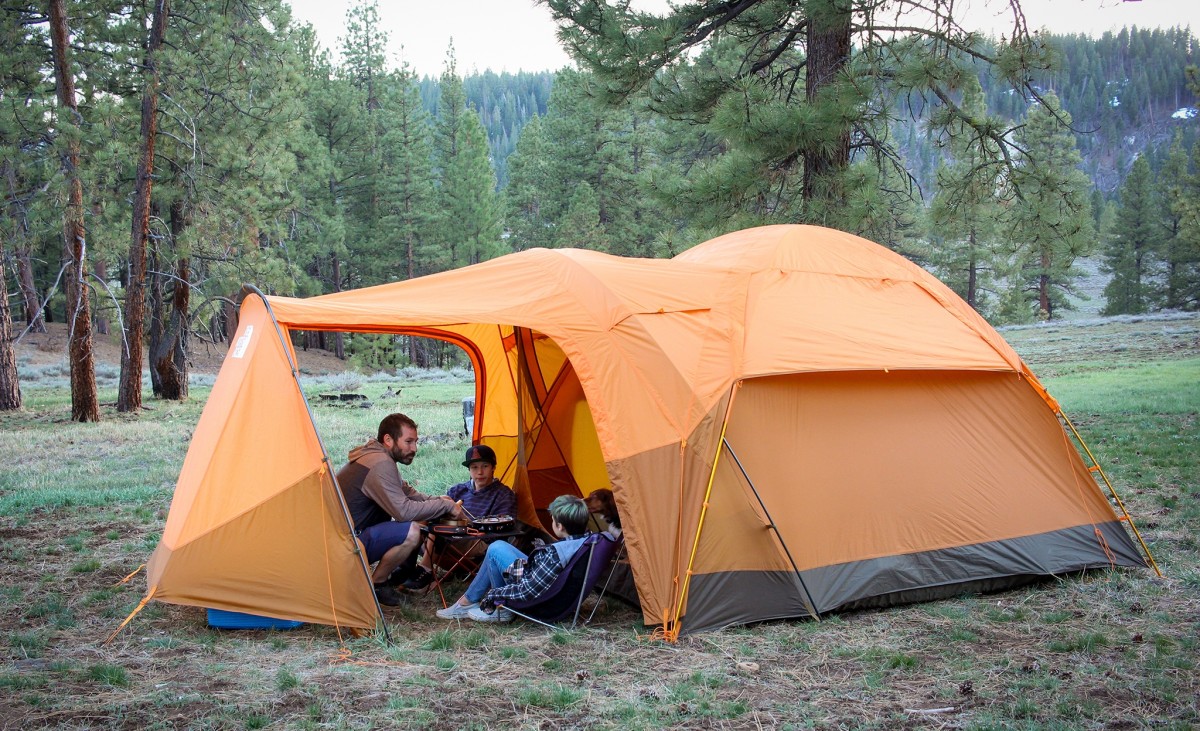In this richly detailed outdoor photograph, a family is enjoying a camping trip amidst a vast forest filled with countless evergreen trees stretching into the background. At the heart of the image stands a vibrant orange and gray tent, partially open to reveal the cozy interior adorned with yellow accents and red-trimmed zipper linings. The man, dressed in a brown sweater and blue shorts, is seen crouching over a cooking pot, likely using an electric burner as there is no visible open flame. Near him, one child, wearing a blue shirt and a black hat with a red logo, sits facing outward, while another child, clad in a blue plaid jacket and jeans, reclines in a fold-out chair. There appears to be a third child, partially obscured, only their head visible. Surrounding the tent are various camping essentials, including what seems to be the bottom of a blue cooler. The family sits on the lush grass, immersed in their camping setup, inside the peaceful expanse of this enormous evergreen forest, capturing a moment of tranquility and togetherness.